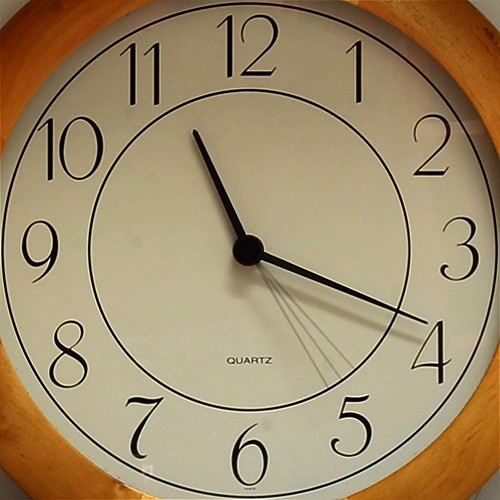This close-up color photo shows a detailed view of a round clock with a wooden frame. The clock face is primarily white, featuring plain black Arabic numerals from 1 to 12 in a classic and clear font. Above the 6 o'clock position, the word "quartz" is inscribed. The clock has three hands: a black hour hand, a thin black minute hand, and a gray second hand. The minute hand is approaching the numeral 5, indicating a time of approximately 11:18 and 23 seconds. Notably, the reflections and shadows of the minute hand create the illusion of multiple minute hands, adding a unique visual effect. Additionally, the face of the clock displays two concentric blue circles, with the blue-lined numbers positioned between them. The corners of the photo frame reveal subtle glimpses of the surrounding white wall, further emphasizing the central focus on the clock.